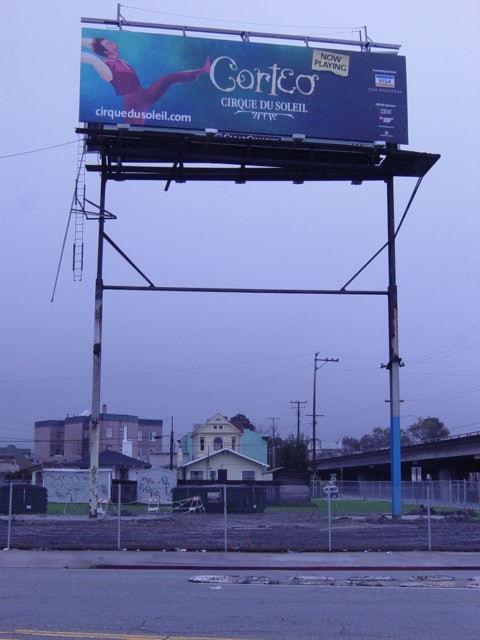The vertical photograph captures a towering billboard viewed from ground level. The imposing structure, estimated to be three to four stories high, is supported by large metallic posts resembling a football field goal post. The billboard is adorned with ladders hanging off its sides, suggesting either damage or maintenance work. The service platform appears slightly tilted, potentially due to the design or recent wear. The billboard advertises "Corteo" by Cirque de Soleil, prominently displaying the website CirqueDeSoleil.com. The text reads "Now Playing" and mentions sponsorship by Visa along with other sponsors. The billboard is set against a backdrop of overcast gray clouds, while in the foreground and slightly beneath the billboard, several buildings, possibly residential homes, can be seen.